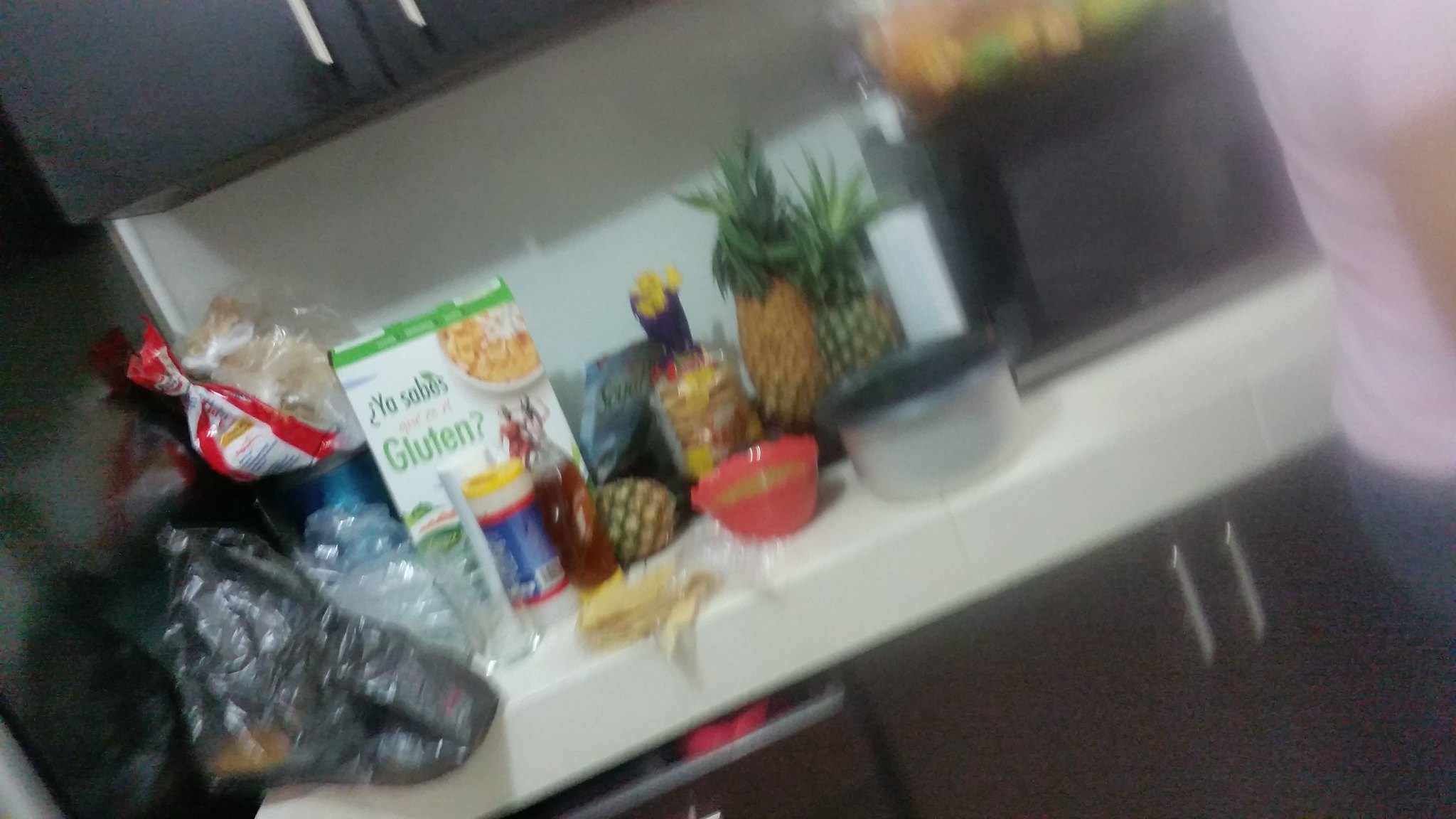The image features a bustling kitchen scene centered around a spacious white countertop cluttered with various groceries and food items for meal preparation. Below the countertop, brown cabinets and a slightly ajar brown drawer on the left are visible, adding a warm touch to the kitchen decor. To the right, a person dressed in a white t-shirt and blue jeans stands, actively engaged in the cooking process.

In the background, an assortment of food items is scattered across the counter. A box of cereal with Spanish text, indicating it is gluten-free, stands out among the groceries. Beside the cereal, three pineapples are noticeable, two upright and one laying on its side. A red bowl containing unidentified ingredients and white Tupperware with a black lid are placed in front of the cereal box, partially obscured by other bottles and containers.

To the far right, a microwave occupies a corner of the counter. On top of the microwave, a clear glass box serves as a makeshift fruit holder, with several lemons neatly arranged inside, adding a pop of yellow to the scene. The overall atmosphere is one of bustling culinary activity, with ingredients and kitchenware scattered in preparation for a meal.